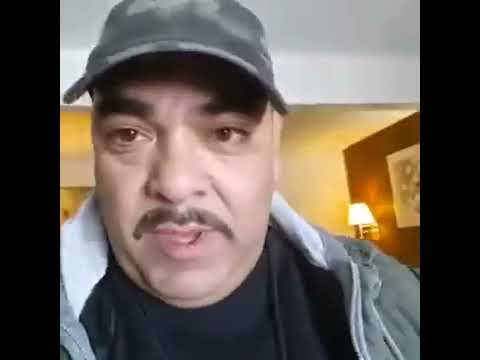The image is a close-up headshot of a middle-aged, stocky man with a double chin and bushy brown mustache. He has warm brown eyes and thick, dark eyebrows, complemented by a gray baseball cap on his head. The man is mid-sentence, his mouth slightly open, looking to his right, away from the camera. He is dressed in a black t-shirt underneath a gray hoodie, visible from the collarbone up. The background reveals a living room with a white ceiling, yellow and brown accented walls, and a light pendant illuminated on the right side. A white portrait is affixed to the wall. The photograph is cropped with black vertical bars on the left and right sides, giving it a letterboxed appearance.